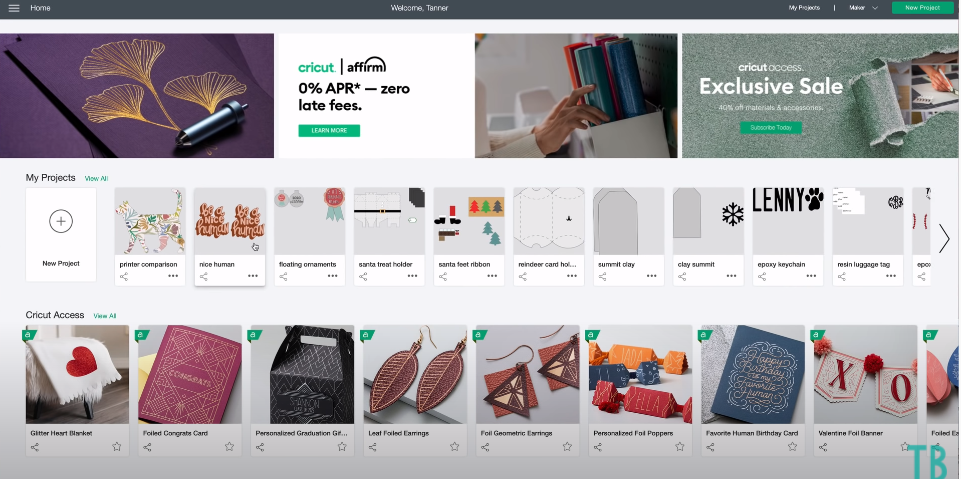Screenshot of a Crafting and Selling Website

This screenshot captures the interface of a website dedicated to crafting, possibly for selling handmade items or for managing creative projects. In the top-left corner, there is a "Home" menu, accompanied by a hamburger icon that users can click to reveal additional navigation options. The top-center of the screen features a welcoming message, "Welcome, Tanner," indicating that the user is logged in. 

To the top-right, there are several actionable options: "My Projects", "Maker", and a prominent green button labeled "New Project". Below these menu items, the screen displays a series of images and promotional banners with accompanying text.

1. On the far left, there is an image of a beautifully designed decorative paper featuring an intricate golden flower pattern.
2. Next to it, a promotional banner for "Circuit Affirm" advertises financing options with "0% APR, 0 late fees," alongside a green button labeled "Learn More."
3. The following image depicts an individual arranging books on a shelf, suggesting perhaps a DIY or organizational project.
4. On the far right, another promotional banner entices users with a "Circuit Access Exclusive Sale" offering 40% off materials and accessories, with a green button for subscribing to this offer.

The repeated mention of "Circuit" throughout the screenshot suggests that this is the name of the website, potentially focusing on crafting tools and materials.